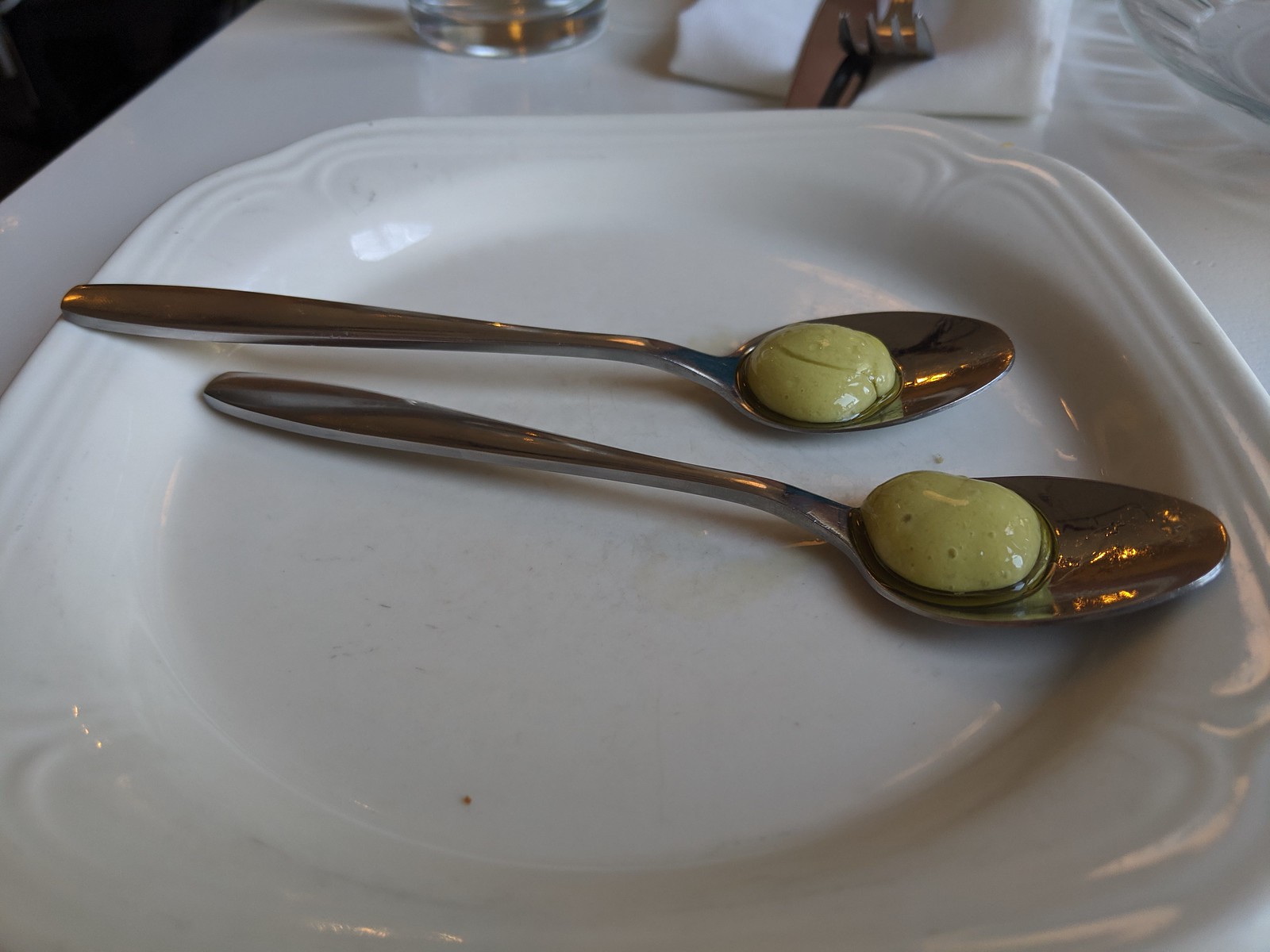This image depicts a neatly arranged dining scene featuring a square white porcelain plate with softened, rounded corners and a decorative rim. The plate, which has a shallow, recessed center, holds two silver-toned spoons positioned horizontally with their handles pointing to the left. On the back part of each spoon, there is a green, textured dollop of a thick, oily substance, perhaps a culinary cream or sauce, forming a small pool of liquid within the spoon. The plate rests on a white linen tablecloth; in the background, the base of a clear glass can be seen alongside a white napkin adorned with a silver butter knife and a four-pronged fork. The overall setting is clean and minimalistic, with a sterile aesthetic that emphasizes the stark contrast between the white, silver, and green elements in the image.